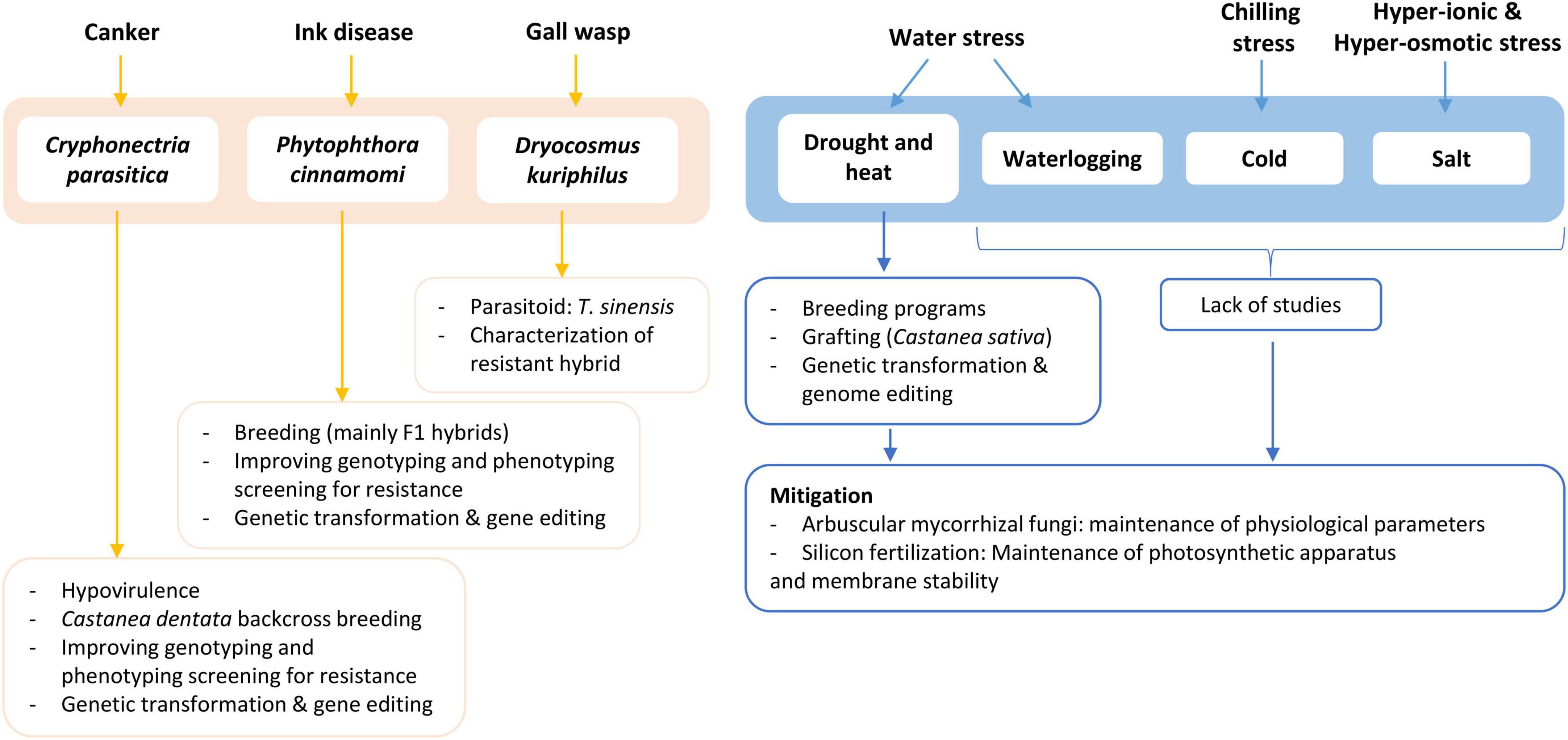The image displays a detailed scientific flowchart on a white background, divided into two main sections with corresponding color schemes and directional arrows. The left section, highlighted in light pink pastel, features three initial terms at the top: "canker," "ink disease," and "gall wasp." Yellow arrows descend from these terms into a pink box containing scientific names: "Cryphonectria parasitica," "Phytophthora cinnamomi," and "Dryocosmus kuriphilus," indicative of biological entities like parasites or diseases. 

On the right section, the flowchart is colored in light blue pastel, starting with terms such as "water stress," "chilling stress," and "hyperionic and hyperosmotic stress." Blue arrows guide from these terms to a blue box with further descriptors including "drought and heat," "water logging," "cold," and "salt." Each arrow on this side delineates specific environmental stress factors affecting ecological conditions. This flowchart offers detailed scientific insights into the relationships and effects of various biological stresses and diseases.